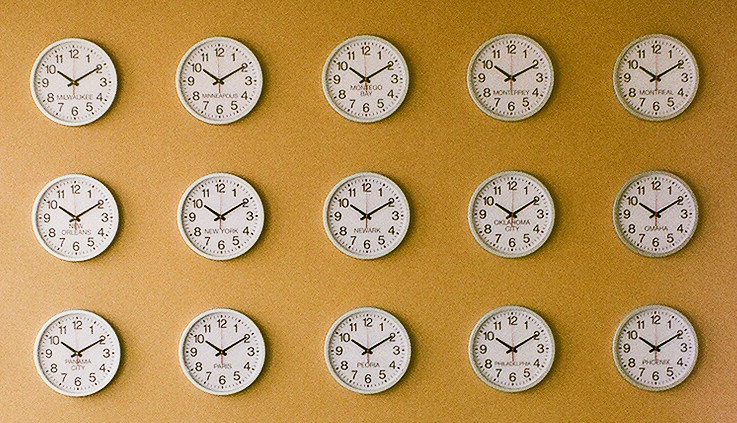The photograph captures a rectangular wall adorned with 15 identical white clocks featuring black numbers, meticulously arranged in a grid pattern of 3 rows by 5 columns. Each clock prominently displays the names of different cities, including Milwaukee, Minneapolis, Montego Bay, Monterey, Montreal, New York, New Orleans, Newark, Oklahoma City, Omaha, Panama City, Paris, Peoria, Philadelphia, and Phoenix. Set against an orange-gold background, every clock is uniformly set to the time 10:10, highlighting an intriguing synchronization across various time zones. The exact alignment and the repetition of the same time on all clocks add a visually compelling element to the image.